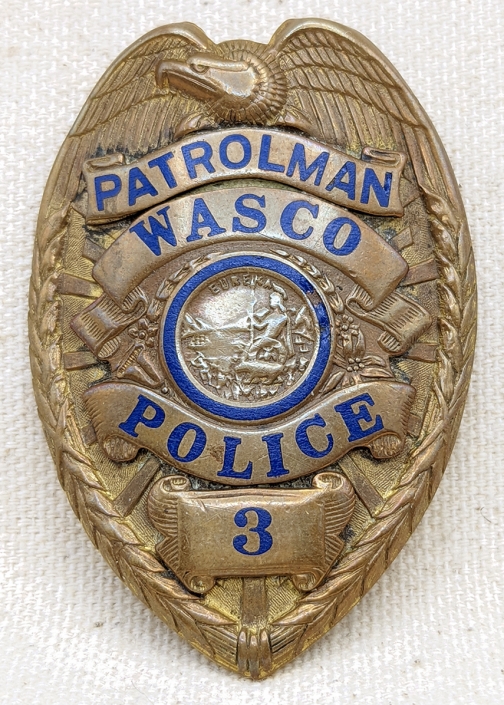The photograph is of an oval-shaped patrolman's badge with a light gold, almost dirty yellow, hue. The badge, set against a white canvas or tissue paper background, prominently features an eagle at the top, with its detailed wings extending out to the sides. The text on the badge is in blue and reads from top to bottom: "Patrolman Wasco" on wavy lines, with "Police" and the number "3" beneath. Enclosed within a blue circle in the center of the badge is the word "Eureka," along with a detailed image of a man on a chariot, appearing to grab something with a claw. Around him, smaller figures, including one with an axe, ascend a hill towards the main character. A thin line resembling lightning descends from above in the scene. The intricate design elements and blue trimming on the badge's center coin-like image provide a striking focal point.